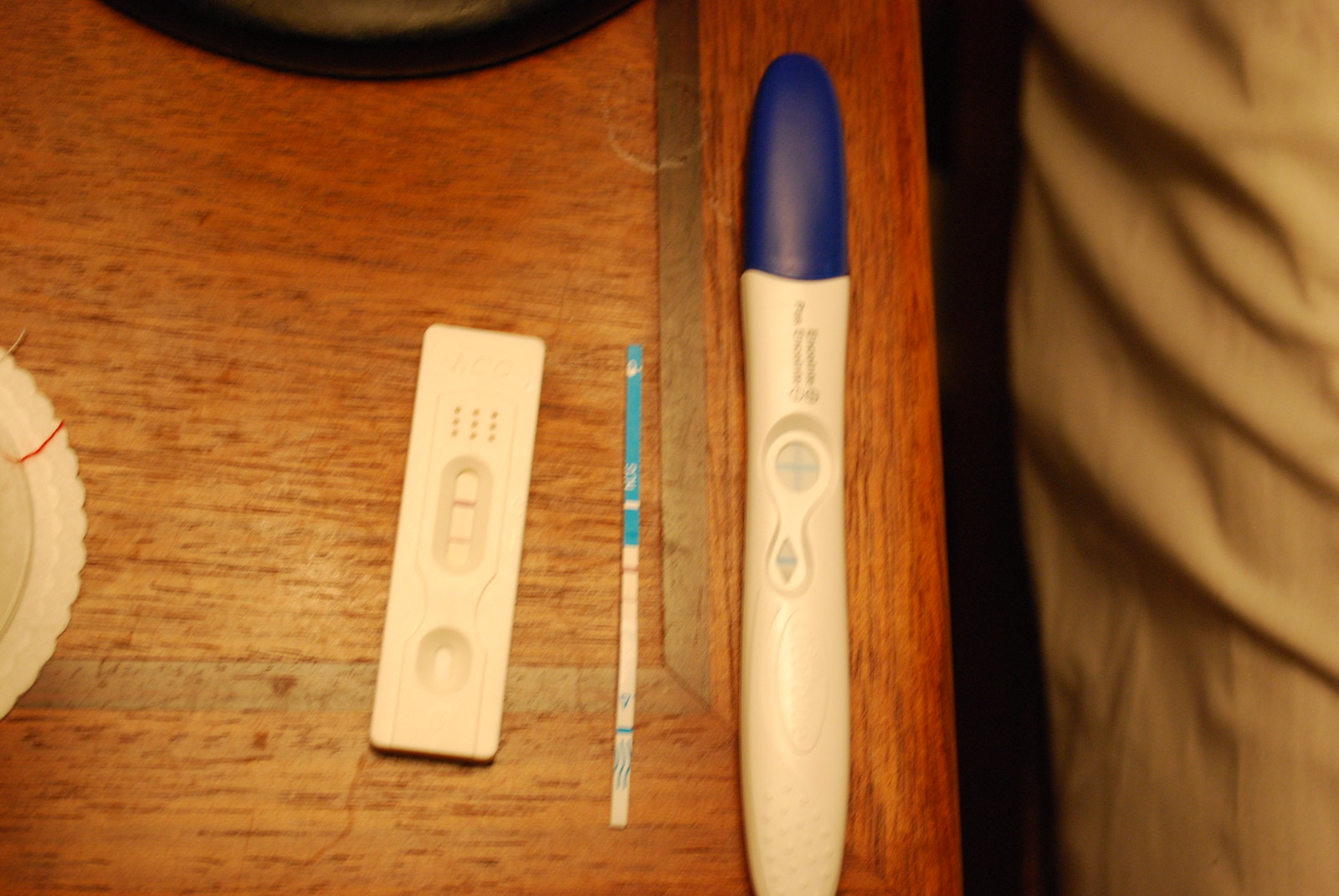A heartwarming photograph captures three different pregnancy tests resting on a wooden nightstand. The nightstand, displaying a few water rings but otherwise in good condition, sits beside a bed with visible linen forming a cozy background. Each test tells its own story: the leftmost one, likely a budget option, shows a red control line and a pink test line, indicating a positive result. The middle test features a delicate design with a prominent red control line and a faint test line, suggesting early detection and barely-there confirmation. The test on the far right, probably from a well-known brand like Clearblue, displays a clear blue plus sign in the window, affirming the positive result with certainty. This trio of tests, ranging from faint to unmistakable, showcase a moment of initial uncertainty turned into joyous confirmation.